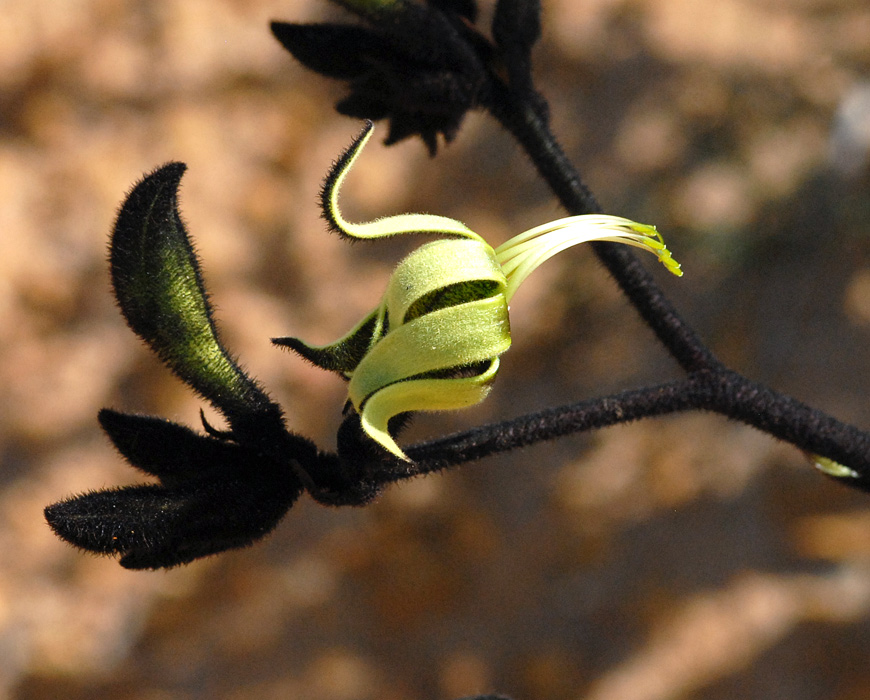This image showcases a close-up of a striking Australian wildflower known as the black kangaroo paw. Dominated by a very dark purple to black stem and coated with black, hair-like trichomes, the plant adds a unique contrast to its vibrant green flower, bud, and leaves. Centered in the image is a pod resembling an opened banana peel, with light green hues and stems protruding from the middle, suggesting the site of nectar or pollen production. The surrounding leaves and stems also carry this unusual black, almost burnt appearance, intensifying the visual impact of the bright green flower. The background is deliberately out of focus, featuring brown splotches that provide a subtle, earthy canvas, further accentuating the distinct and lively colors of the plant.